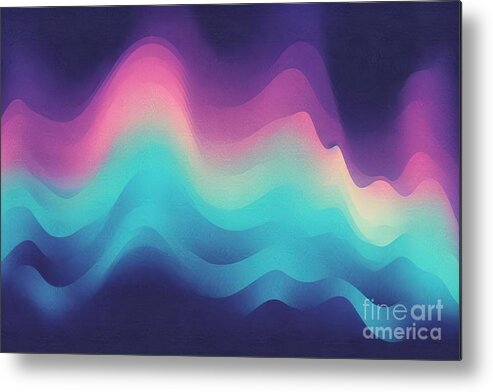The image depicts an abstract wall art print featuring a gradient of multicolored waves on a canvas, starting from a deep, dark purple at the top. As the waves flow downward, they transition through various vibrant colors: from pink to peach, merging into a yellow wave, followed by teal or turquoise, then light blue, and culminating in a dark indigo wave towards the bottom. The waves are layered in a pattern reminiscent of a rainbow spectrum, with delicate blending between each shade. The background of the waves maintains a rich indigo hue, adding depth to the composition. In the bottom right corner, the artwork is titled in white lowercase letters as "Fine Art America." The print appears to be hung on a white wall, enhancing the contrast and visual appeal of the colorful waves.